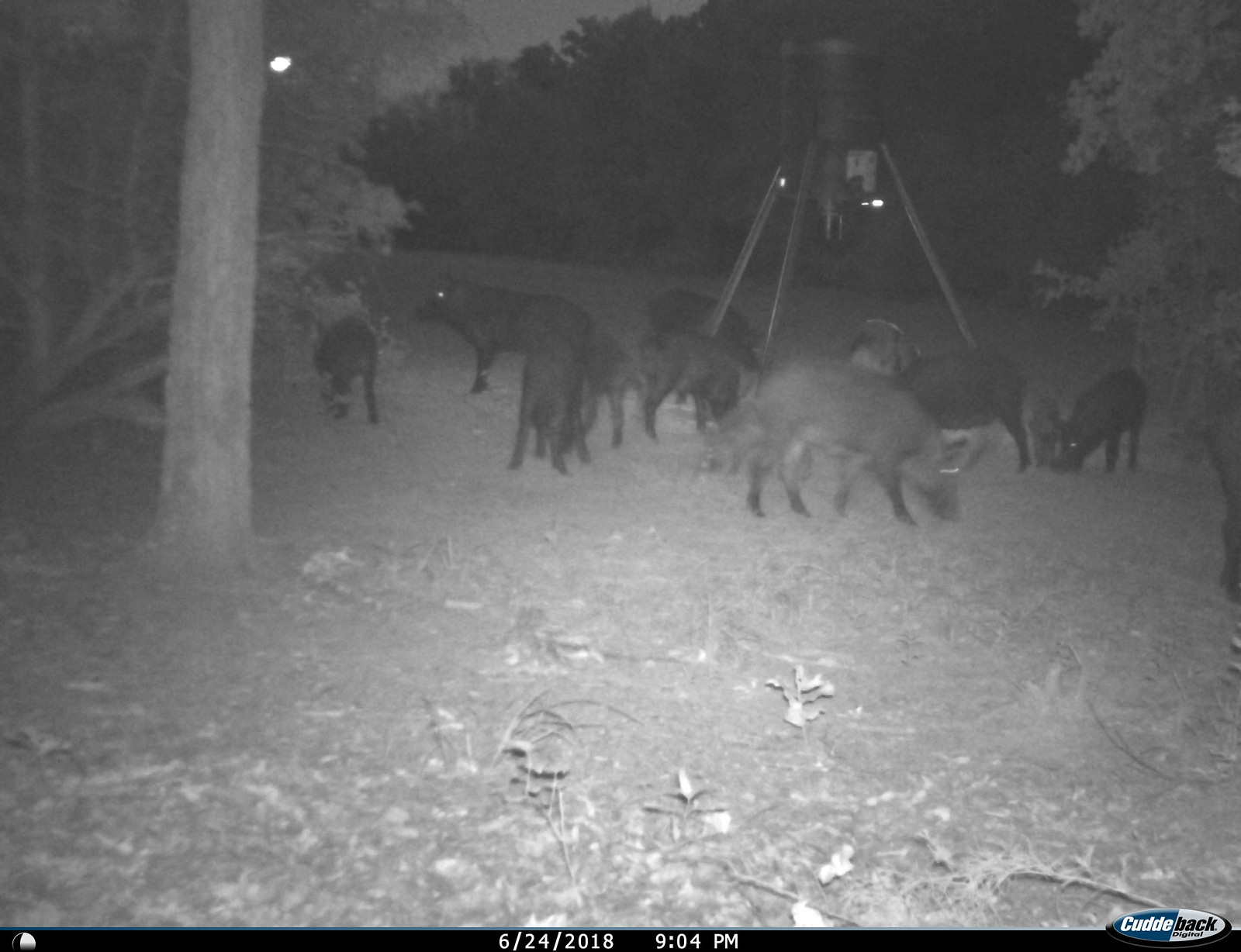This black and white photograph, taken on June 24, 2018, at 9:04 p.m., captures a nocturnal scene in an open field lined with tall evergreen trees. The image shows a group of dark-colored pigs, possibly mistaken for other animals, as they gather around a feeding area, likely beneath a feeder or a cylindrical drum setup on a tripod. The field, covered in grass, brush, and sticks with scattered leaves and tree trunks, appears to be illuminated by lighting possibly attached to the tripod structure. In the background, the moon can be seen shining through tree branches, adding a subtle glow to the scene. The bottom right of the image shows a circular logo, half blue and half gray, with the brand name "Cuddle Back" indicated in contrasting text.